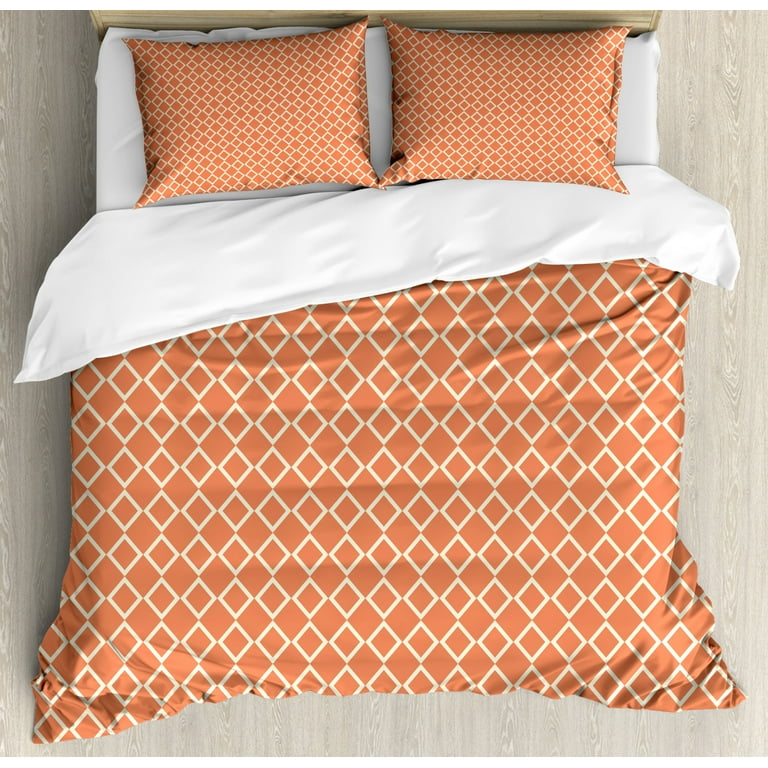The photograph is a detailed, full-color aerial view from above, capturing a neatly made bed positioned on a light gray, wood-planked floor. The square image, likely taken indoors under artificial light, showcases a subtle, barely visible wooden headboard at the top. The headboard matches the floor's grayish-off-white wood texture. The bed features two orange pillows and a comforter predominantly orange with intricate white diamond patterns that interconnect at their points. The comforter's top portion is folded down, revealing its white underside and underlying white sheets. The diamonds on the comforter have white outlines with solid orange interiors, creating a striking geometric design consistent across the entire bedspread.